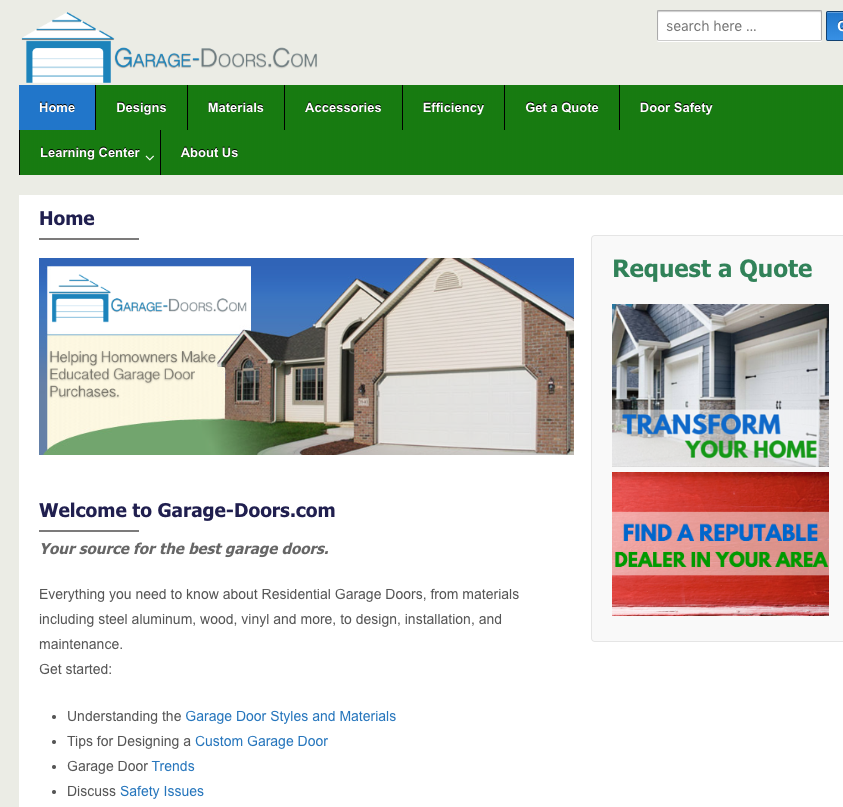**Landing Page Overview for GarageDoors.com**

The landing page for GarageDoors.com features a clean and organized layout with a light gray background border. The centerpiece of the page is a white space with various sections and links. 

**Header:**
- **Top Left Corner:** A blue and white image of a garage with a white door outlined by blue lines and borders. Above the garage door is a pyramid-shaped, three-level structure.
- **Logo:** Positioned to the right of the image, the text "GARAGE-DOORS.COM" is displayed in uppercase letters, with "GARAGE" and the hyphen in blue while the rest is in gray. The initial letters "G" and "D" are larger than the rest.
- **Top Right Corner:** Features a white search bar with the placeholder text "search here..." in gray.

**Navigation Bar:**
- **Leftmost Section:** A blue tab with "HOME" written in white.
- **Adjacent Sections:** Seven tabs against a dark green background with white text, labeled: "DESIGNS," "MATERIALS," "ACCESSORIES," "EFFICIENCY," "GET A QUOTE," and "DOOR SAFETY."
- **Additional Sections:** A second row with two sections, "LEARNING CENTER" and "ABOUT US", separated by vertical bars.

**Main Content Area:**
- **Upper Left Corner:** The section title "HOME".
- **Image:** A mixed media picture-illustration of a house with a garage door, accompanied by the same logo from the header.
- **Welcome Message:** Below the image, the text: "Welcome to Garage-Doors.com" and in italics, "Your source for the best garage doors."
- **Informational Text:** Three lines of introductory text followed by bullet points; the last bullet point highlights "discuss safety issues" where "safety issues" is in blue and the rest in gray.

**Sidebar:**
- **Box on the Right:** A gray portrait-oriented box.
  - **Green Header:** "REQUEST A QUOTE".
  - **Image:** A picture of various garage doors attached to homes with the caption, "Transform your home."
  - **Text:** Instruction to "Find a reputable dealer in your area."

This descriptive overview captures the layout, color scheme, and textual information provided on the landing page for GarageDoors.com, offering a comprehensive and detailed understanding of the site’s design and content elements.